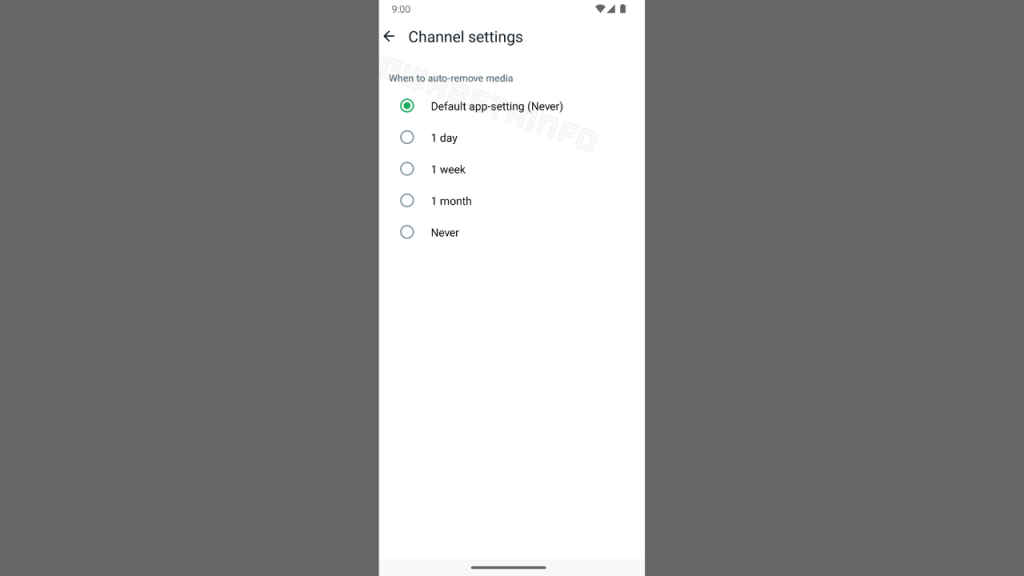The image prominently features a smartphone screen displaying a settings menu against a mostly gray background, with lighter gray shades on the left and right sides. The middle section of the image is dominated by a white rectangular strip running vertically. 

At the top left of this white strip, the time is displayed in black as "9:00," along with a black Wi-Fi symbol, a fully black reception bar indicating strong network reception, and a fully filled battery icon. Below this, the text "Channel settings" appears in black, accompanied by a left-pointing arrow.

Further down, amidst a grayish-blue section, there is a heading in black text reading, "When to auto-remove media." Below this heading, five circular radio buttons are arranged vertically, each representing a different selection option. The first option, which is selected and indicated by a green highlighting circle, reads "Default app-setting (never)" in black text. The subsequent options are "1 day," "1 week," "1 month," and "never," all in black text and listed in descending order.